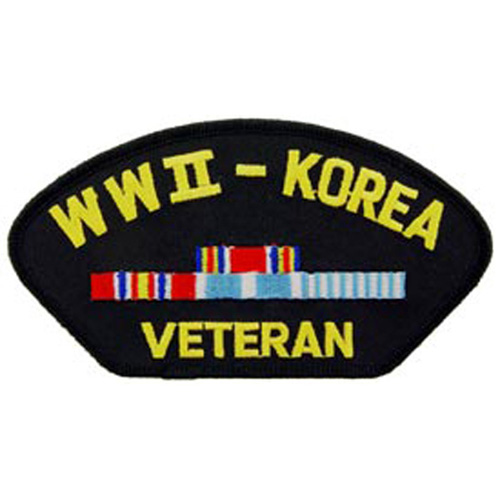The image features a black badge, shaped similarly to a mushroom cap or a shell, designed for a veteran's military uniform. This patch has prominent yellow text curved across the top that reads "WW2-Korea" and "Veteran" at the bottom. The text is all in capital letters. The center of the badge is adorned with two horizontal rows of colorful lines. The shorter top row has a pattern of red, yellow, blue, white, red, yellow, blue, white, red, and blue. The longer bottom row, closer to the "Veteran" text, features a sequence that includes red, white, blue, white, red, yellow, red, white, blue, white, red, repeating across its length. The detailed color bands add a vibrant contrast to the otherwise solid black patch, giving it a distinguished and recognizable appearance.